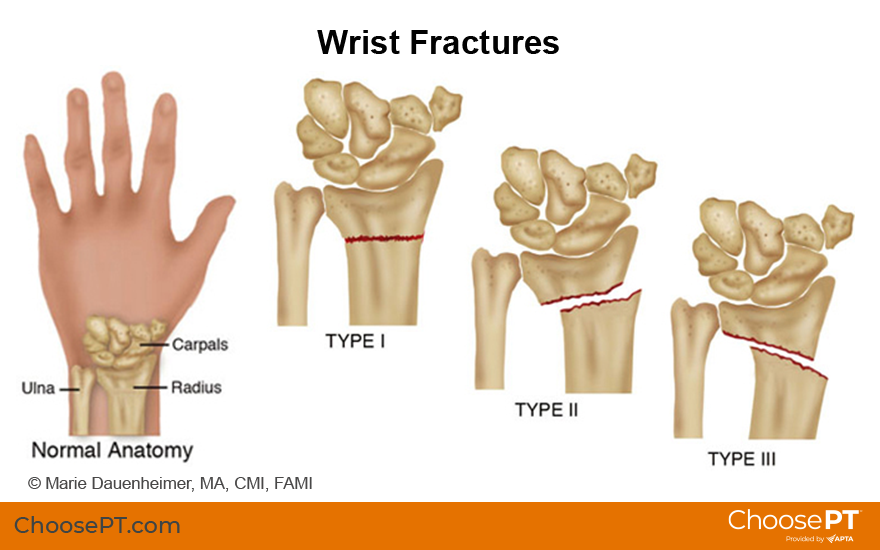This detailed diagram illustrates different types of wrist fractures against a white background. The primary image on the left shows a hand, palm side down, with bones overlaid. Key anatomical labels include 'ulna' on the bottom left of the wrist, 'carpals' at the upper right, and 'radius' on the bottom right. The label "Normal Anatomy" is displayed prominently in bold black letters at the bottom of the hand illustration.

Adjacent to this, three additional diagrams, angled downwards to the right, depict types of wrist fractures. Each fracture type focuses on the radius bone. Type 1 fracture has a red line indicating a break at the top portion of the radius. Type 2 shows a more severe break with the radius split in half and slightly shifted to the left. Type 3 fracture displays an even more pronounced separation of the bone fragments. 

At the bottom left corner of the diagram, the illustration is credited to Marie Dauenheimer, MA, CMI, FAMI. An orange banner runs along the bottom of the image, bearing the website choosePT.com on the left, and the phrase "choose PT provided by APTA" on the right alongside a business logo.